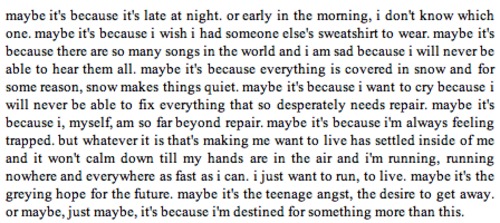The image depicts a scan or screenshot of a densely packed black text on a white background, reminiscent of a journal entry. The text flows in straight horizontal lines, exploring a deeply introspective and melancholic narrative. It begins with the uncertainty of time, contemplating whether it’s late at night or early in the morning. The words capture a yearning for comfort through the metaphor of wearing someone else's sweatshirt and an underlying sadness about the innumerable songs that will remain unheard. It reflects on the stillness that snow creates and the profound sense of despair over the irreparability of some aspects of life, including the writer's own perceived brokenness. The text conveys an intense feeling of being trapped and a restless urge to live fully by running aimlessly yet passionately. It contemplates the flickering hope for the future intermingled with teenage angst and an intrinsic belief in a destiny that surpasses the current discontent.